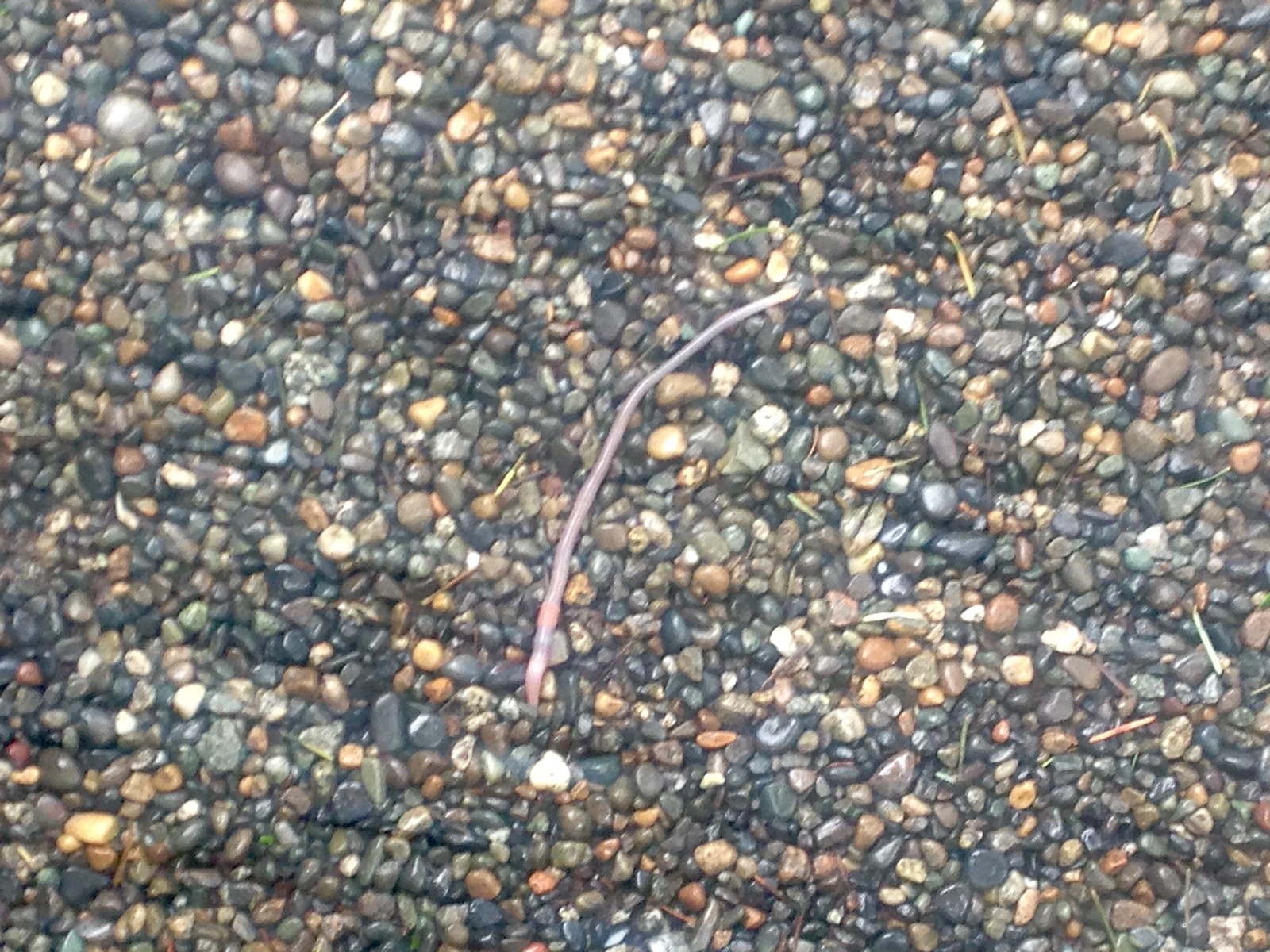This vibrant daytime photo provides a top-down view of a thin, pink earthworm stretched out vertically at the center of a diverse and colorful gravel bed, possibly wet and shiny, giving the illusion of being submerged in a shallow body of water. The gravel consists of various small rocks and pebbles in multiple hues, including black, brown, white, orange, green, and gray, creating a visually intriguing mosaic. These pebbles are smooth and lie directly next to each other, some appearing almost translucent under the light. Scattered amongst the gravel are pieces of grass and a few twigs, contributing to the natural setting. The worm, prominently positioned, contrasts sharply against the multicolored backdrop, with its light brown or tan body and slightly pink-tinted head seemingly navigating through an enchanting, miniature landscape.